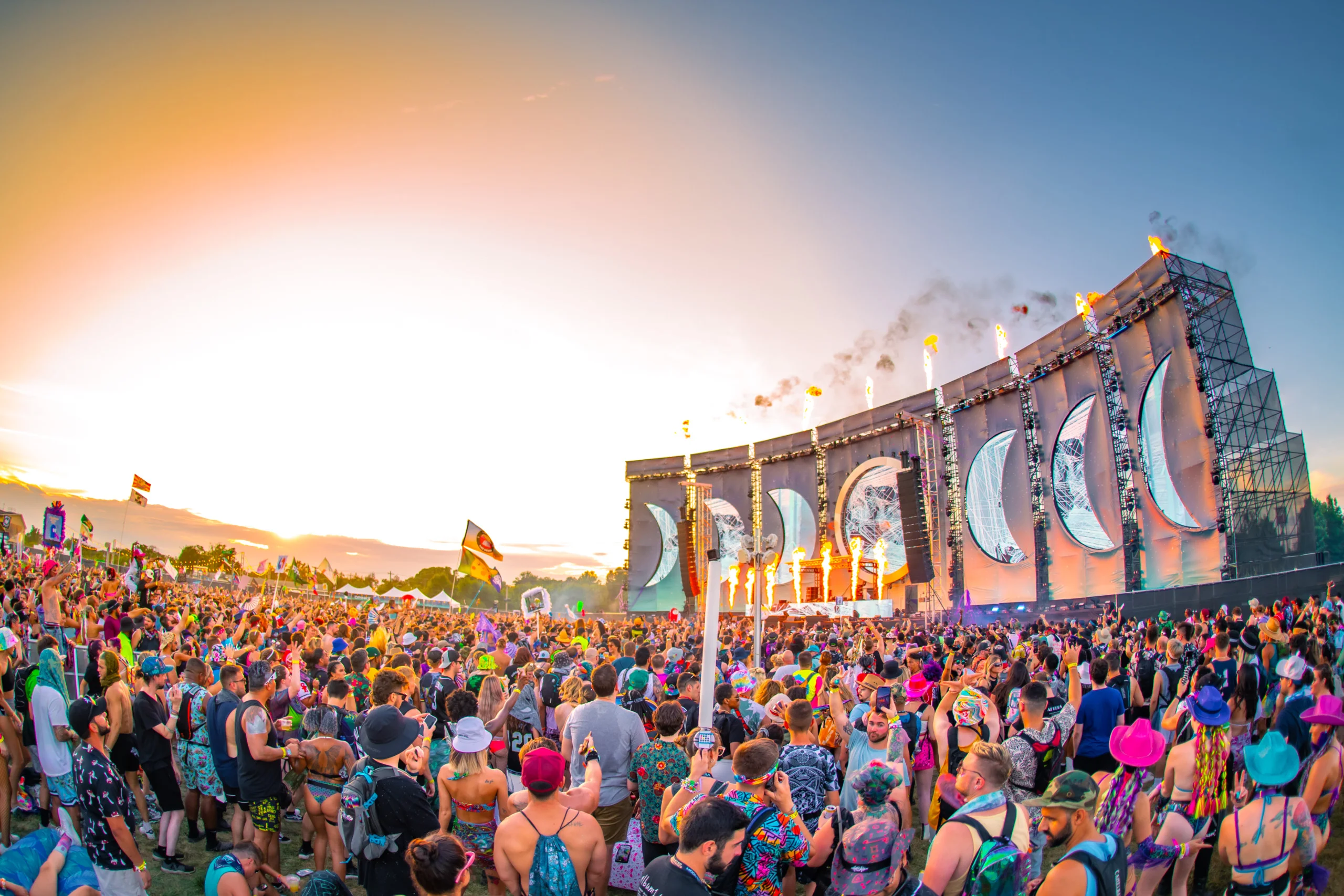The image depicts a lively outdoor festival during summertime, featuring a large crowd oriented towards a stage. The vibrant crowd is dressed in brightly colored, neon clothing, with many donning neon pink and blue cowboy hats, swimsuits, halter tops, and sleeveless shirts. A few attendees carry backpacks. The stage is a striking temporary structure of black scaffolding adorned with fabric illustrations depicting the phases of the moon, with a prominent full moon at the center and crescent moons on either side. Flames shoot up impressively both from the top and the base of the stage. Yellow banners and a long curved gray wall frame the scene, with the wall itself also decorated with moon phases. There is a noticeable glare from the setting sun on the left-hand side, suggesting the festival is transitioning into the evening as the crowd enjoys the performance.